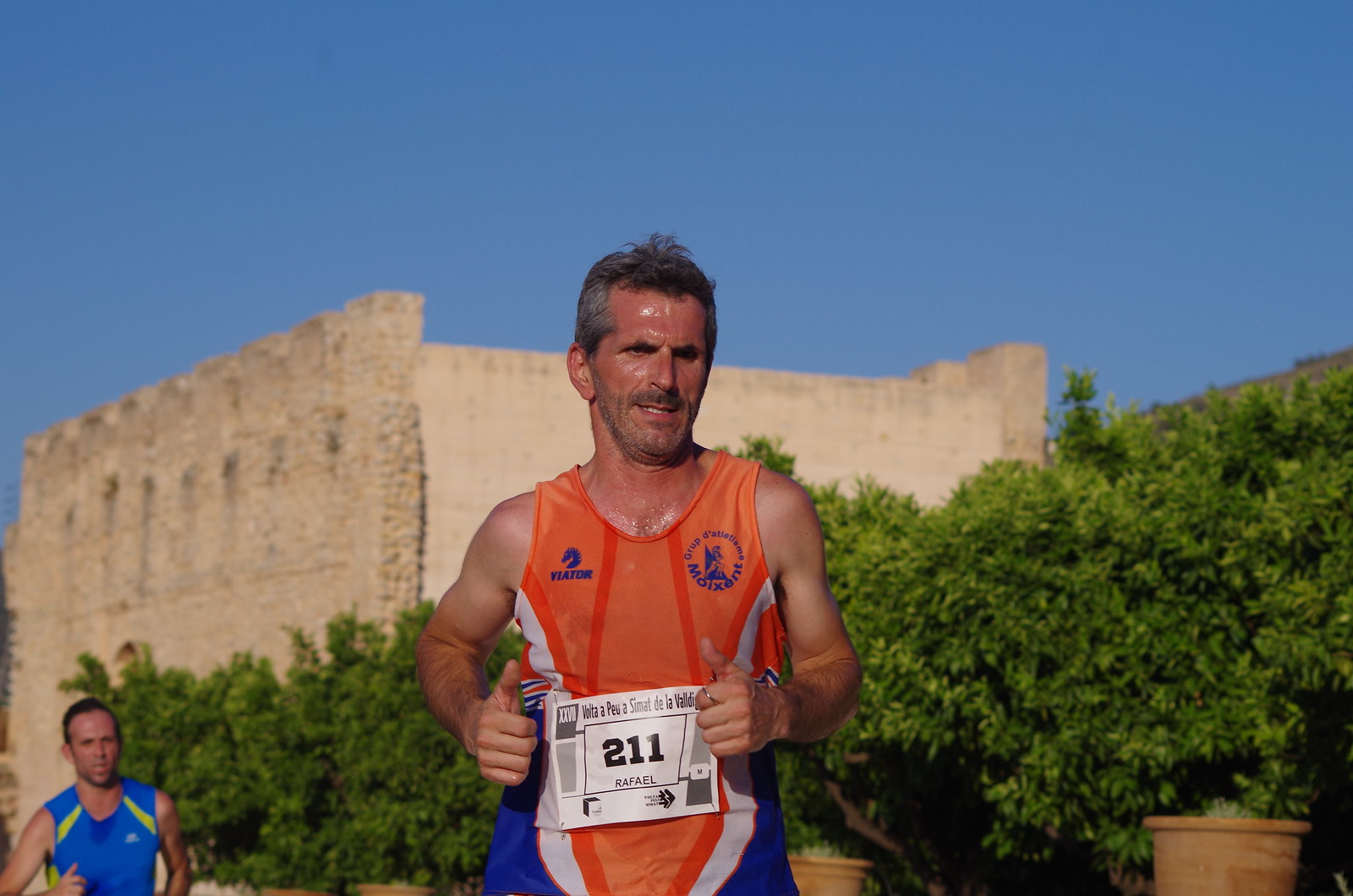The image captures a dynamic scene of a runner, Raphael, wearing the number 211 on a white race bib that also displays the Roman numeral "XXVII" and some unreadable text in a different language. He's clad in an orange shirt with "Yeeter" and possibly other text, and blue, orange, and white shorts. Raphael is running at a steady pace, clearly exerting effort as his sweat-soaked shirt clings to his fit frame. Behind him, another runner is visible, dressed in a blue shirt with yellow trim, also displaying sweat stains prominently around the neck area. The backdrop features lush greenery, including trees and bushes, and a stone brick structure or fort, suggesting a scenic and possibly historic race location bathed in daylight without a cloud in the sky.